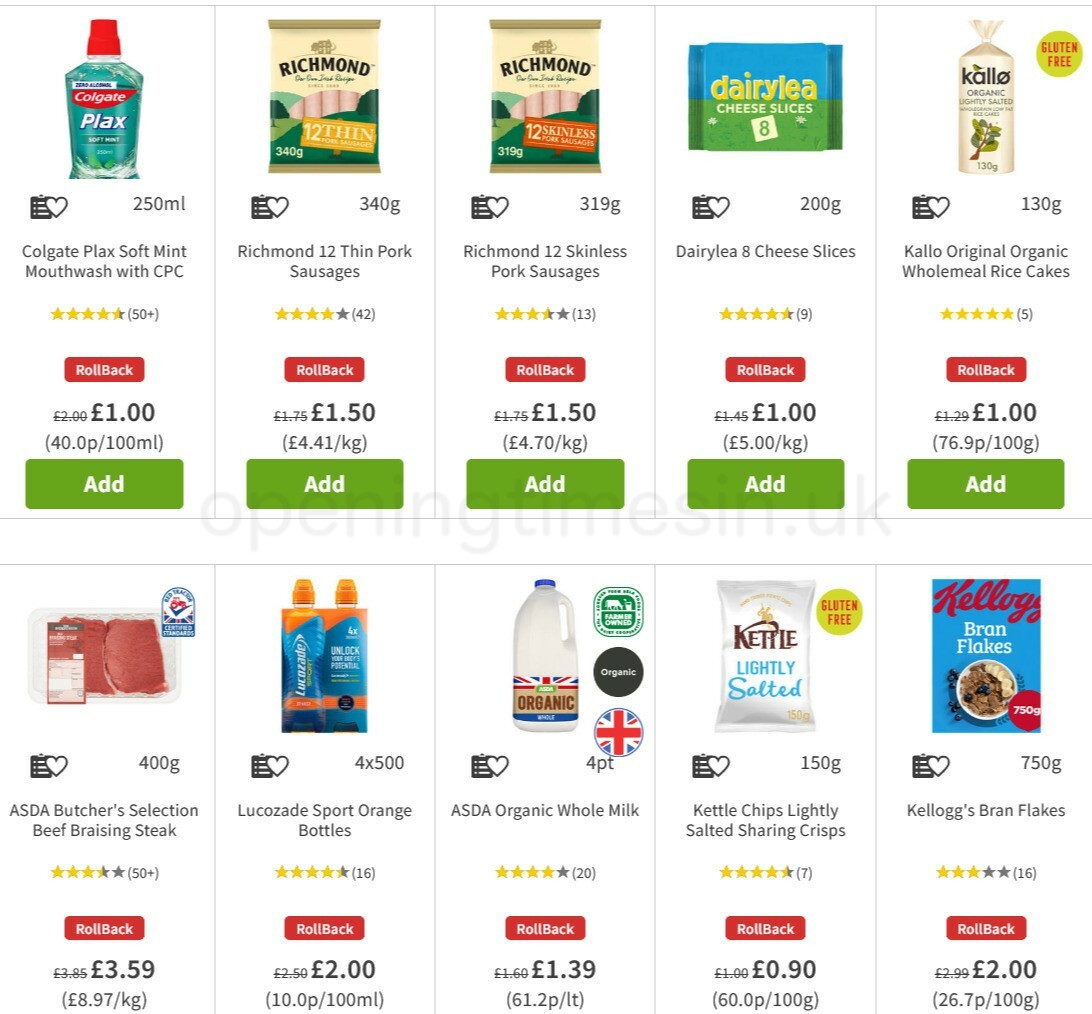This advertisement showcases a variety of discounted products from a store, with notable reductions on popular items. Colgate Soft Mint Mouthwash is now available for £1, down from £2. Thin Pork Sausages are priced at £1.50, reduced from £1.75. Cheese slices can be purchased for £1, previously costing £1.45. Rice cakes are on sale for £1, reduced from £1.29. Kellogg's Frosted Flakes are now £2, down from £2.99. Lightly Salted Sharing Crisps are priced at £1, a reduction from £1.90. Whole Milk is on offer for £1.39, down from £1.60. Lucozade Sport Orange Bottles feature a rollback price of £2, reduced from £2.50. Lastly, the Butcher's Selection Beef Braising Steak is now £3.59, down from £3.85. These significant discounts are part of Walmart’s rollback prices in the UK, providing excellent value for customers.